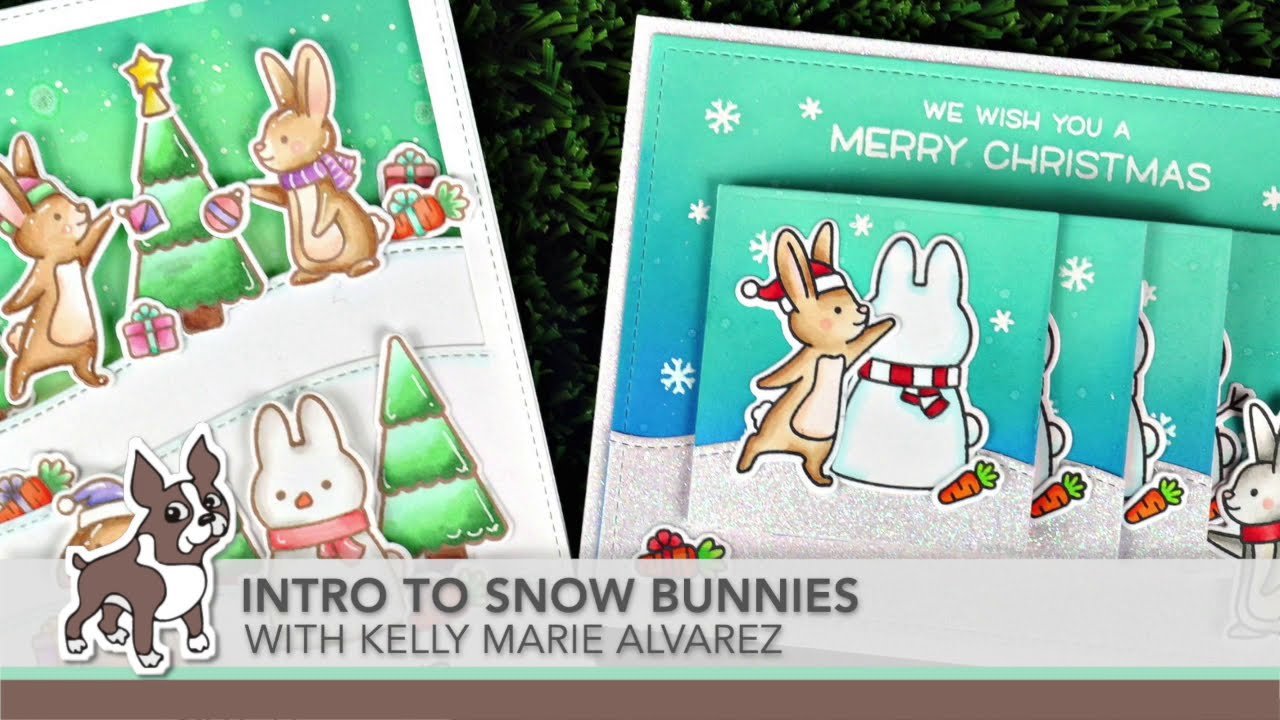The image is a detailed illustration resembling Christmas cards featuring festive scenes with bunnies. On the left side, there is a vertical paper strip showcasing two cartoon rabbits near the top Christmas tree and a white rabbit with a red shawl near the bottom Christmas tree, each tree topped with a star. On the right side, another paper strip illustrates a cheerful scene of a brown animal creating a snowman resembling a rabbit, with a carrot placed nearby, possibly about to be used for the snowman's nose. Above this scene, the text "We wish you a Merry Christmas" is prominently displayed. The background features greenery, mimicking Christmas tree leaves, enhancing the festive atmosphere. At the bottom of the image, there is a light gray horizontal strip featuring a cartoon image of a bulldog on the left and the text "Intro to Snow Bunnies with Kelly Marie Alvarez" on the right. Below this is another horizontal brown strip, adding a contrasting element to the composition.